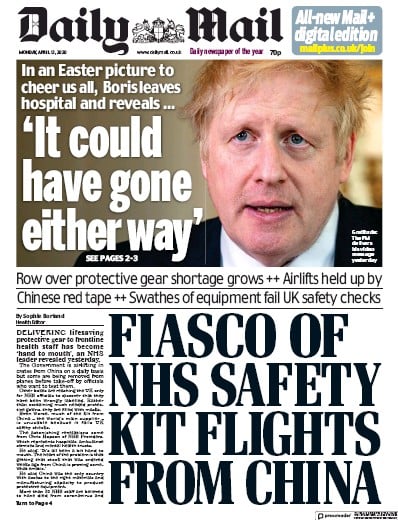This image captures the front page of a newspaper, specifically the "Daily Mail". At the top of the page, the title "Daily Mail" is prominently displayed with a crest situated between the words "Daily" and "Mail". To the right of the title, there is a header indicating "All New Mail Plus Digital Edition".

The lead story features a photograph of a man with furrowed eyebrows and messy hair. The headline next to the image reads: "In an Easter picture to cheer us all, Boris leaves hospital and reveals ...". Below this headline, a quote in quotation marks states, "It could have gone either way (see pages 2-3)."

Further down, the front page addresses growing concerns about a shortage of protective gear with the subheading: "Row over protective gear shortage grows," followed by bullet points highlighting additional issues:
- "Airlifts held up by Chinese red tape"
- "Swaths of equipment failed UK safety checks"

In large bold print, the headline "Fiasco of NHS Safety Kit Flights from China" dominates the page.

To the left of this main headline, there is a block of very small text, consisting of eight paragraphs, that is too tiny to read. For further details on the story, a note in bold print directs readers to turn to page 4.